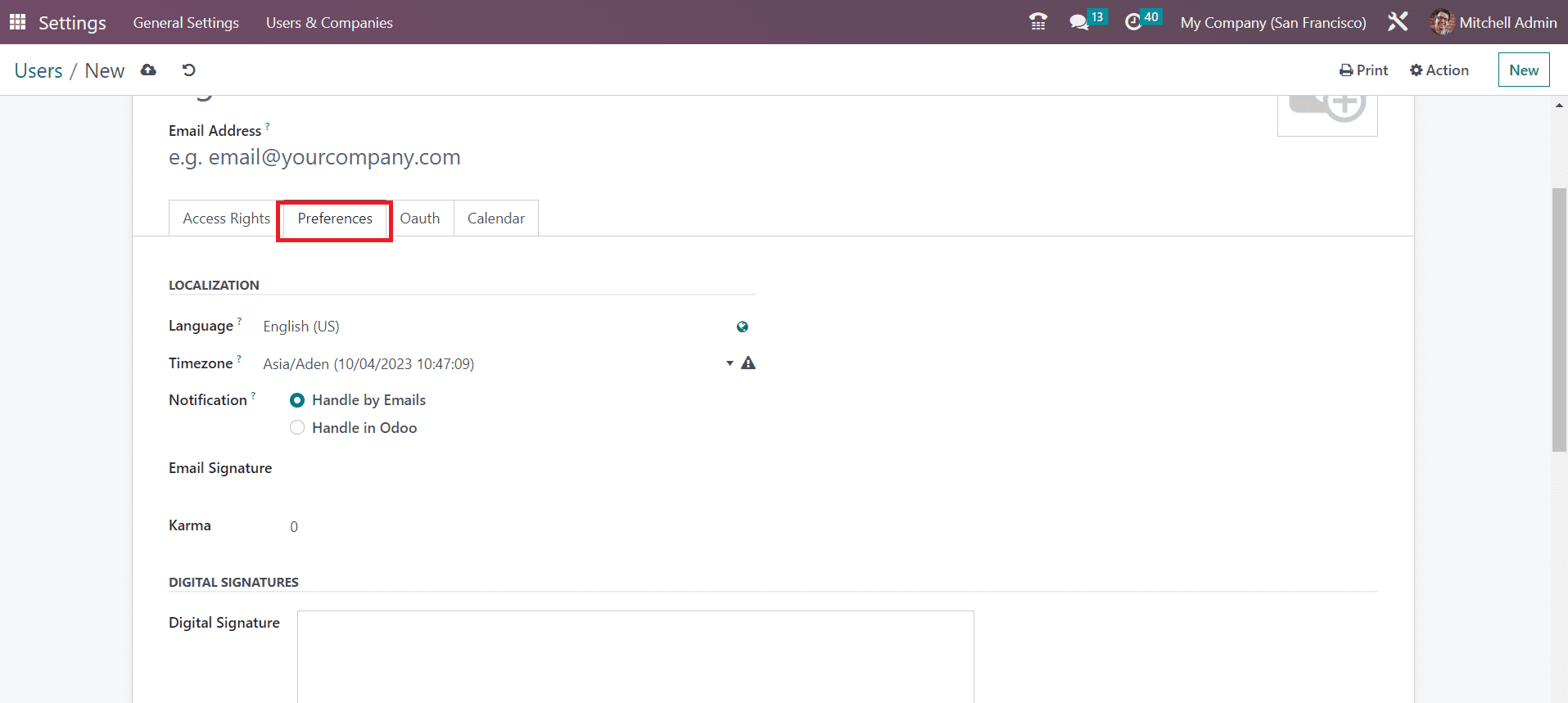Screen capture of a computer screen displaying a settings interface. At the top of the screen, there is a maroon-colored bar labeled "Settings," with subcategories such as "General Settings" and "Users and Companies." Further to the right, there are additional options including "My Company," "On Air," "In San Francisco," and "Prince's and Mitchell Administration," accompanied by thumbnail images of the respective users or administrators.

Below the main bar, the screen section labeled "Users / New" provides further options such as "Print," "Other Actions," and "New." The page is scrolled slightly, cutting off the very top. The first visible field is for entering an email address, with an example displayed as "email@yourcompany.com." Below this field, there are various settings options including "Access Rights," "Preferences" (which is currently selected), "Oath," "Calendar," and "Localization," which is set to "US English." The time zone is configured for the Asia region.

Under the notification settings, email handling is enabled. There are also sections for setting an "Email Signature," "Karma," and "Digital Signatures," which appear to be customizable options for business setup and administration.